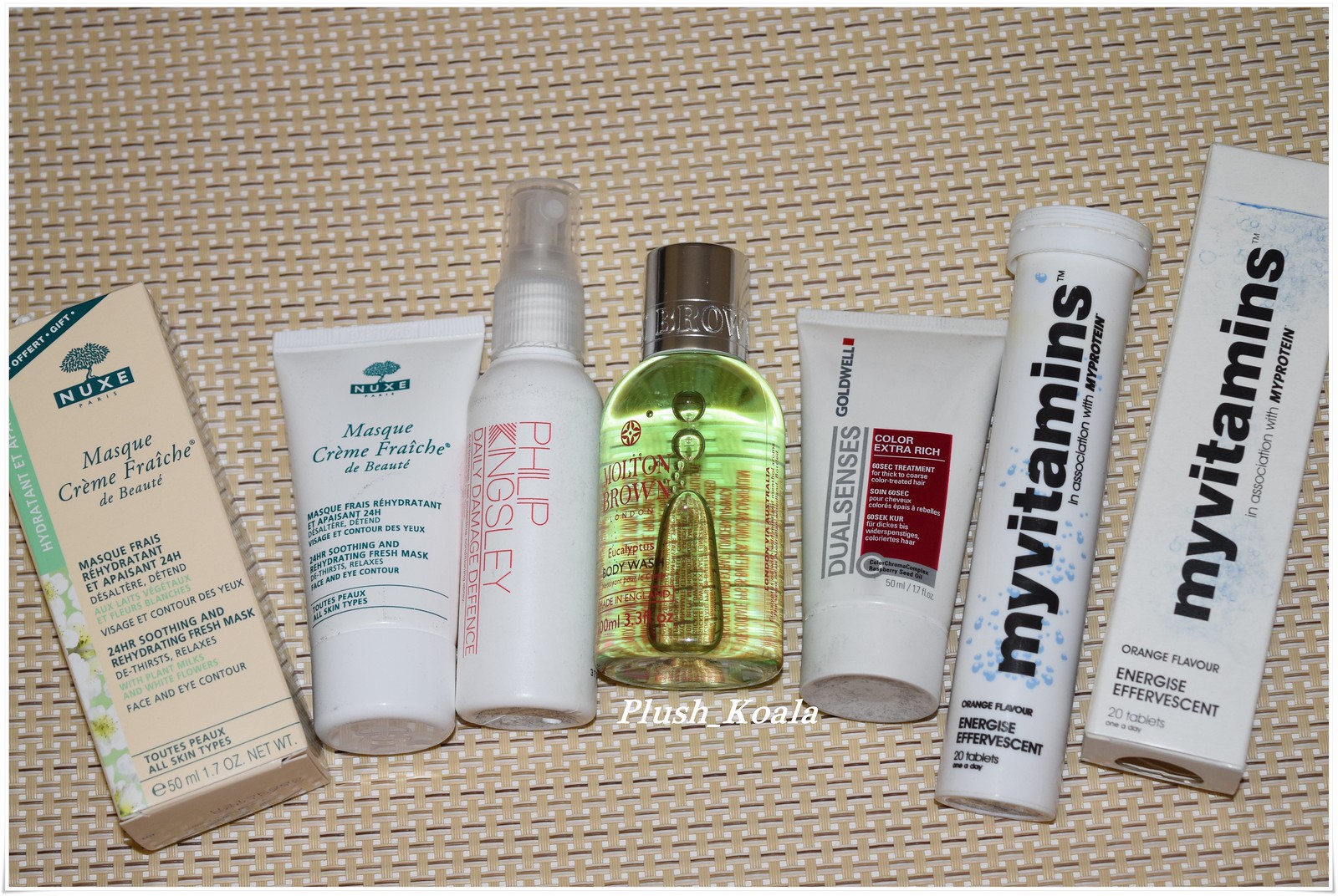The horizontal image captures an array of seven distinct products meticulously arranged on a textured beige placemat adorned with white dots, resembling a woven fabric. 

On the far left, a beige box labeled "Massage Creme Fraiche" in French, accentuated with green and blue text, takes the spotlight. Adjacent to it is a white tube with green lettering, identified as a mask. Beside the mask stands a sleek, white spray bottle, exuding simplicity and elegance. 

Following the spray bottle is a transparent perfume bottle containing a vibrant green liquid. To the right of the perfume, a tube marked with the name "Dual Senses" is placed strategically. Next in line is another white tube, elongated and labeled "My Vitamins." The lineup concludes with a corresponding "My Vitamins" box on the far right, maintaining the pristine white theme. 

The deliberate arrangement and varied designs draw attention to the unique identity of each product against the subtly textured background.